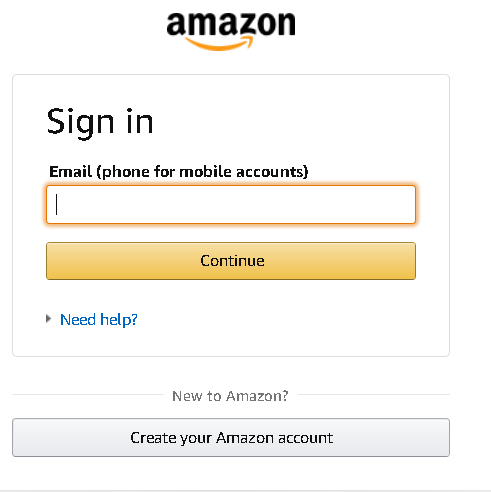This image showcases the sign-in window for Amazon, a leading e-commerce platform. At the top of the screenshot, the Amazon logo is prominently displayed, featuring the word "Amazon" in black with a distinctive yellow curved arrow underneath. The sign-in window itself is primarily white with black text. At the top of this window is the word "Sign-In." Below this, there is a white input field where users can enter their email, phone number, or mobile account details, and a cursor currently positioned within this text box indicates it's ready for input. Directly beneath the input field is a prominent yellow button inscribed with "Continue" in black text.

Further down, there is a blue text link reading "Need help?" with a question mark situated immediately following the word "help." Below this link is a thin gray line that separates the previously mentioned elements from additional options. Centered beneath this line, the text "New to Amazon?" invites new users to create an account. Following this invitation is a light gray rectangular button with the black-text prompt "Create your Amazon account," which encourages new users to register.